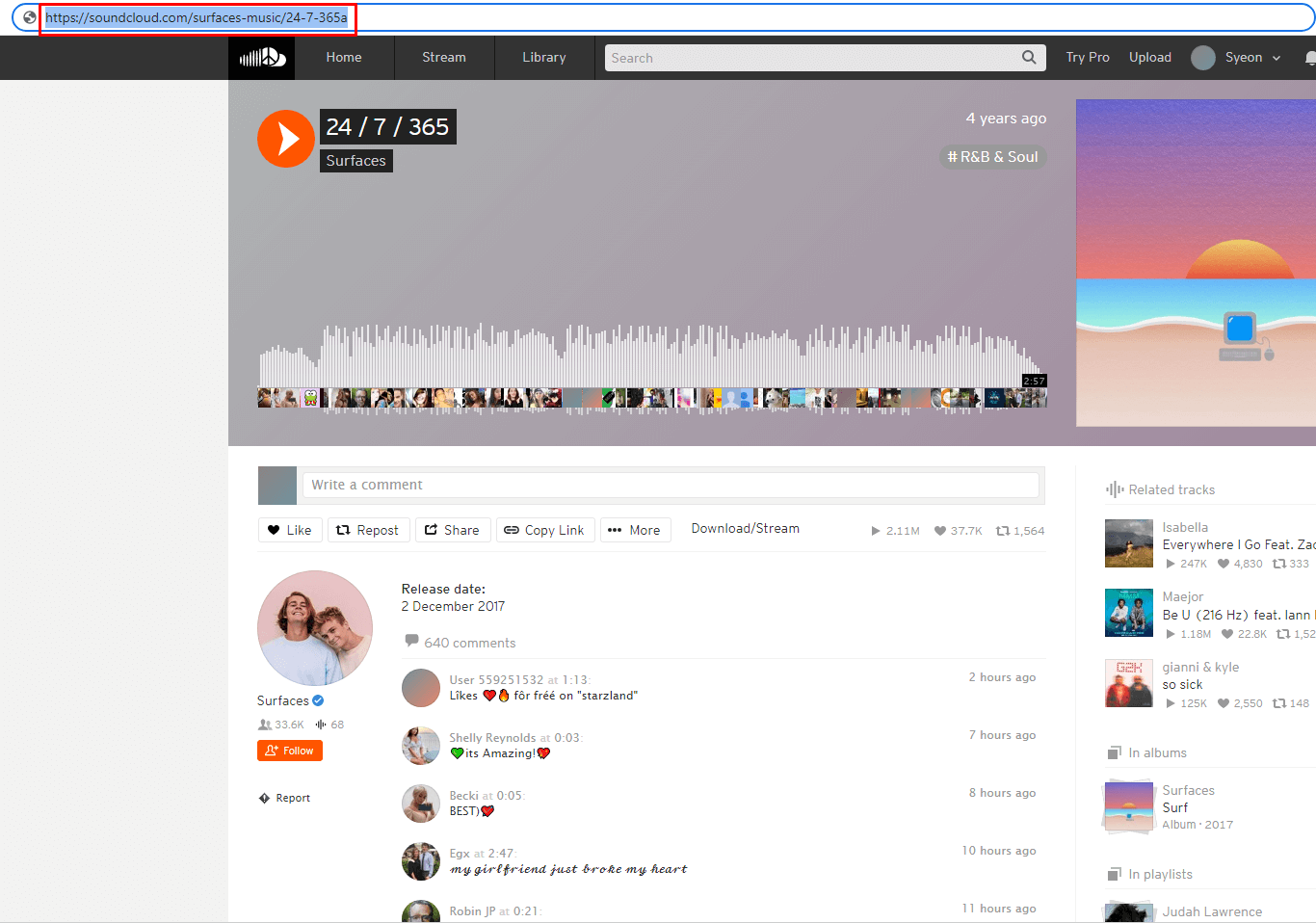This image is a screenshot of a web page from SoundCloud. At the top, the URL is visible, reading "https://soundcloud.com/surfaces-music/24-7-365a," highlighted in blue with black text and surrounded by a red rectangle, while the URL bar itself is outlined in blue.

The webpage header features the SoundCloud logo on the upper left, which is a white cloud icon. To the right of the logo are navigation tabs labeled "Home," "Stream," and "Library," along with a search bar. Additional tabs labeled "Try Pro" and "Upload" are also present, followed by a user icon and the username "Scion."

The main section of the page showcases a play button next to the title "24-7-365." Below the title, the artist’s name "Surfaces" is displayed. Further details reveal that the track was posted four years ago and is categorized under the hashtag "R&B & Soul." The page also includes stylized sunset graphics and a bar showing different user icons at the bottom of this top section, with status bars indicating how many times users have listened to the song.

Below this section is a comments area where listeners can leave their thoughts and feedback on the track.